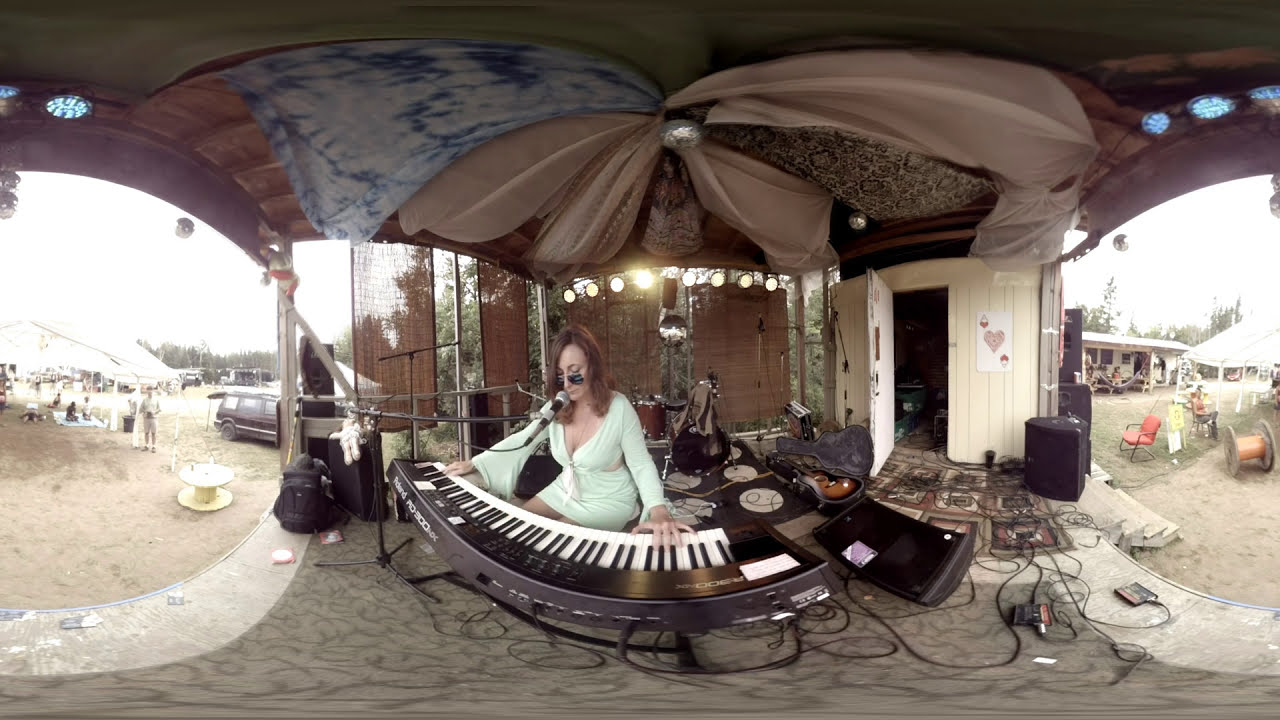In this panoramic image, a woman sits playing a long, curved keyboard that appears to be positioned on a patterned gray carpet. She is dressed in a deep-cut, flowing white dress with long sleeves and has shoulder-length brown hair, wearing sunglasses and a microphone positioned near her mouth. Surrounding her is an intricately decorated tent-like structure with fabric draped from above, converging towards the center in a flower-like design, featuring various shades of color. To the left and right of her, you can see speakers connected by numerous wires scattered on the floor. 

To the left of the scene, a white sunshade roof shelters a few seated and standing people. Further out, you notice parked cars and an additional pavilion. To the right, there’s a walkway next to another pavilion, a large spool that may contain wire, a building, and a seat placed outside. In the background, there are more people and another spool, contributing to the busy atmosphere captured in this detailed snapshot.